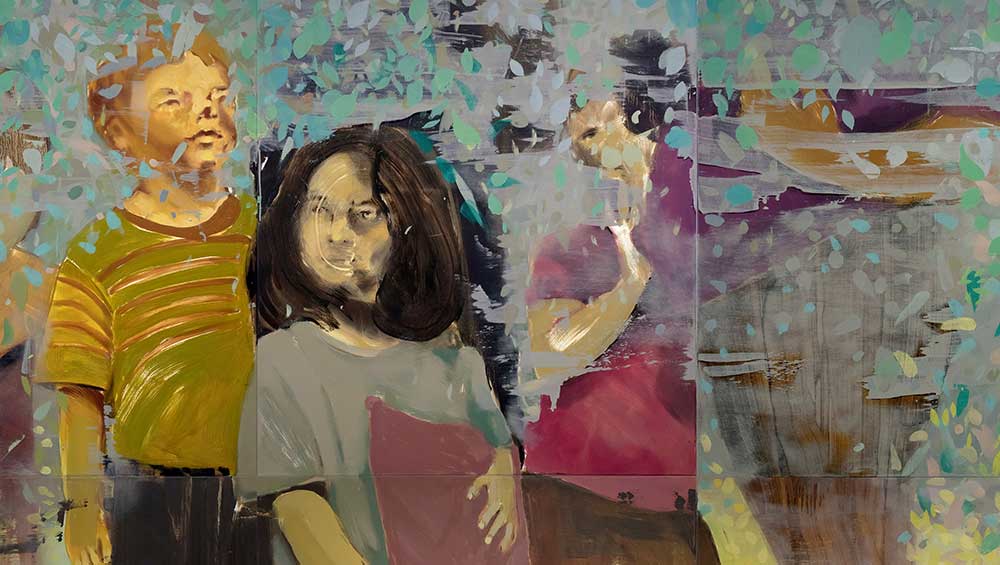The artwork appears to be a watercolor or digitized painting featuring three children centrally positioned against a colorful background with varying shades of green and yellow. On the left, a boy with yellowish skin tone and short hair is depicted looking upwards. He wears a yellow and brown short-sleeved shirt paired with black pants. In the middle, there is a girl with brown hair that falls to her neck and is parted at the side. She has a lighter yellow complexion, and she is dressed in a lighter gray-blue shirt while holding a violet-colored pillow in her left hand. To the right of her, another individual is partially obscured by the background's green leaves and brown spots. This person is wearing a violet-pink shirt but is less defined compared to the other two figures. The background consists of abstract, blended colors, enhancing the painting's ethereal and dreamy ambiance. There is no text associated with the image.